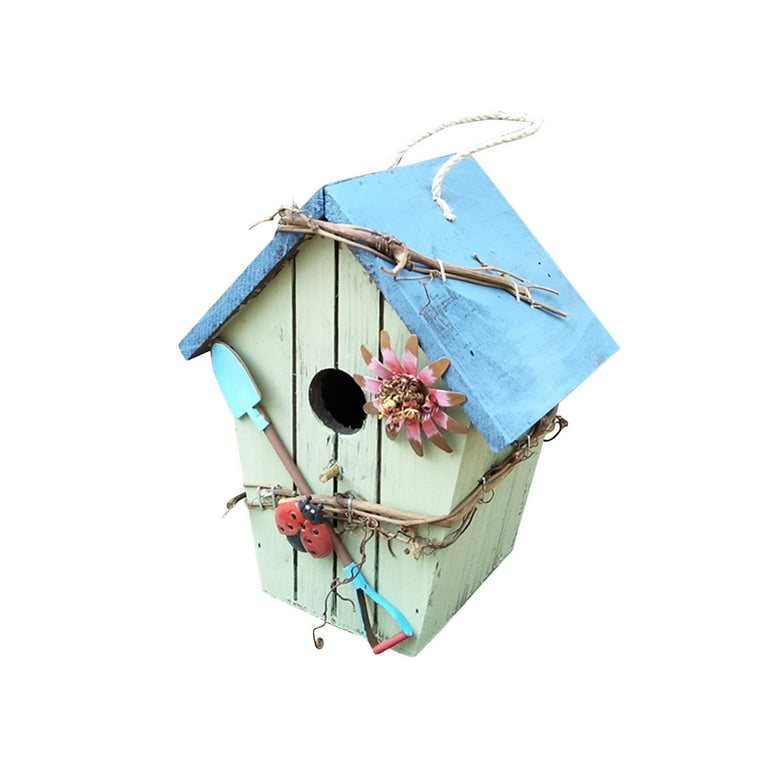This close-up image features a handmade wooden birdhouse set against a stark white background. The birdhouse showcases a pastel design with a light blue, triangular slanted roof adorned with a small gray twig and a white rope stapled at the center, presumably for hanging the birdhouse. The sides of the birdhouse are painted a soft pastel green. Prominently displayed on the front, there's a circular entrance hole, where birds can enter, and beneath this hole a few carved ridges or lines are visible.

To the right of the entrance hole, a pink and yellow flower adds a touch of vivid color. Diagonally crossing the front face from the top left to the bottom right is a blue shovel, partially wrapped in twine, which ends at a red and black ladybug perched near the bottom. The birdhouse's charming and detailed decor, including its ornamental twig and shovel, floral accents, and warm color palette, makes it a quaint and whimsical addition to any garden or outdoor space.